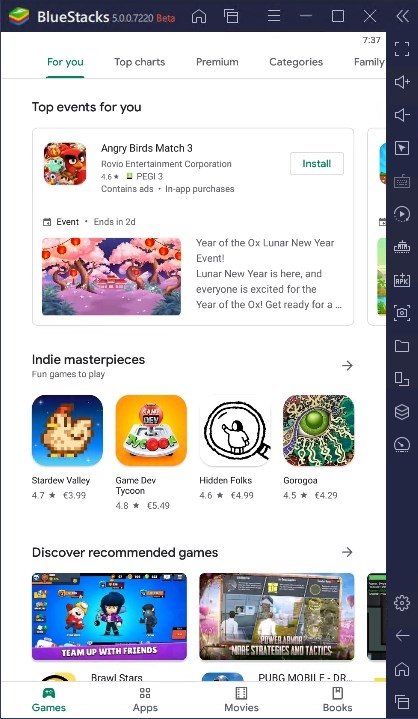This image is a detailed screen capture of the BlueStacks app, showcasing its interface on a mobile operating system in portrait mode, characterized by its taller-than-wide display. The screen has gray banners with control buttons located along the top and right sides, while a white banner at the bottom offers navigation options for games, apps, movies, and books.

The central section of the screen presents a white background with black text, accompanied by several small icon images representing various games. At the top of this section, Angry Birds Match 3 is prominently featured. Below this, there is a recommendation list titled "Indie Masterpieces," showcasing four games: Stardew Valley, Game Dev Tycoon, Hidden Folks, and Gorogoa. Further down, under the "Discover Recommended Games" heading, there are several rectangular-shaped icons for popular games like Brawl Stars and PUBG Mobile.

The BlueStacks branding is visible in the upper left corner alongside their logo, identified as BlueStacks 5.00.7220 Beta. This detailed layout indicates the app's role in facilitating access to various mobile games and applications through its interface.